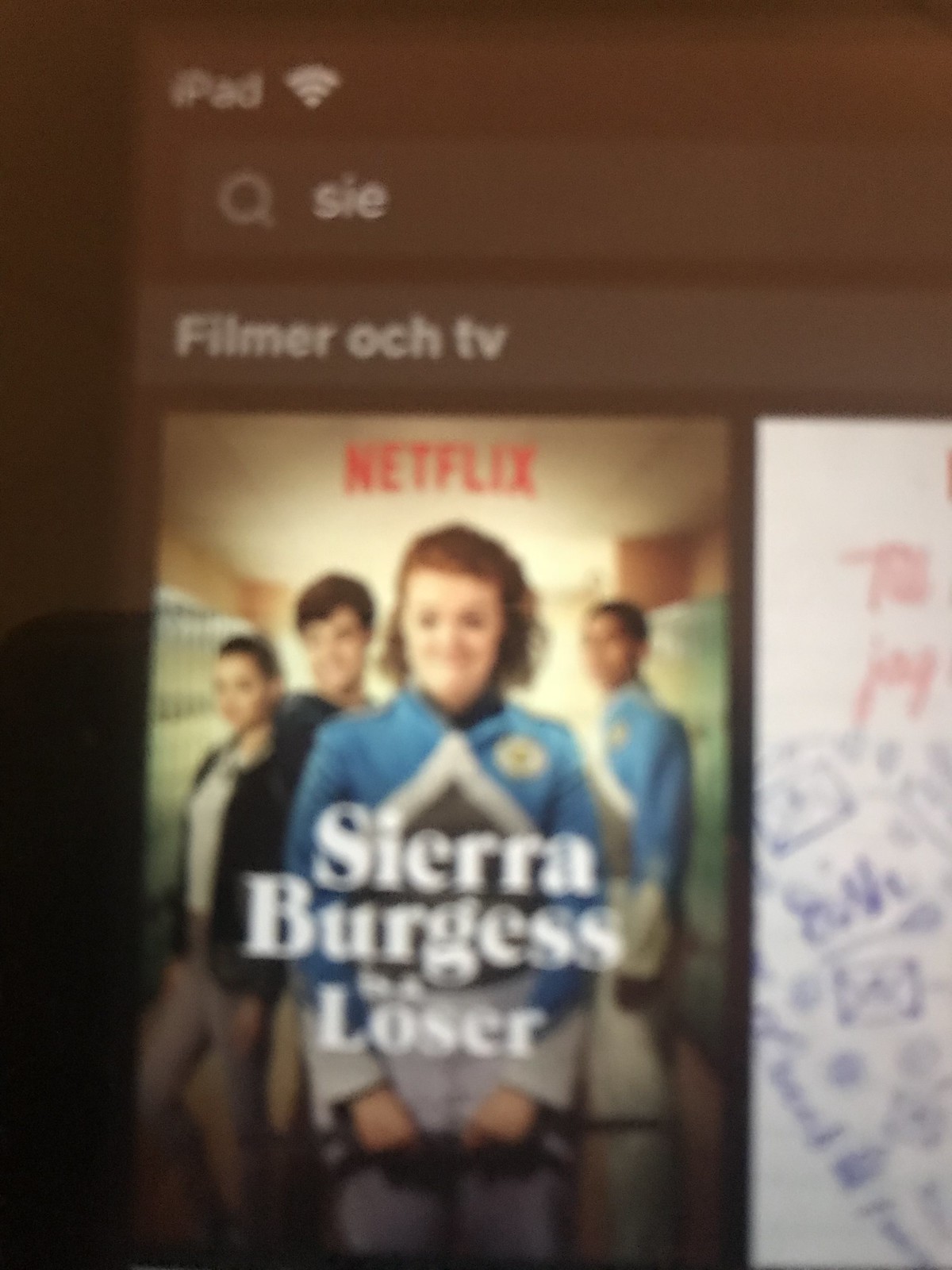The image displays a Netflix interface showcasing the movie "Sierra Burgess Is a Loser." In the search bar above, "S.I.E." is entered, indicating a search for this specific film. The text "Filmer AUKTV" appears near the search bar. The background of the interface is predominantly brown with a black section on the left side. The cover art for "Sierra Burgess Is a Loser" features a Caucasian female protagonist standing prominently in the front, with three other individuals (two males and one female) positioned behind her. Adjacent to this movie cover, there is another movie poster with a white background and red lettering.